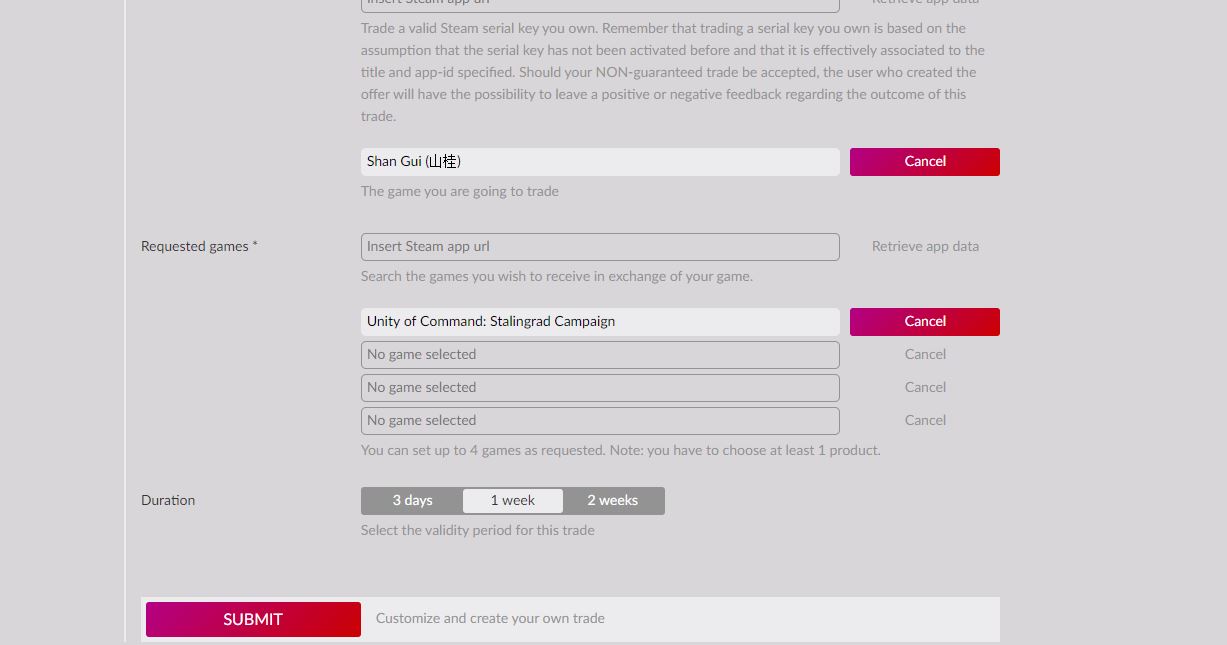Screenshot of a website form used to trade valid STEAM serial keys. The top of the form features an instruction: "Trade a valid STEAM serial key you own." It notes that the trade assumes the serial key has not been previously activated and is correctly associated with the specified title and app ID. If a non-guaranteed trade is accepted, the user who created the offer can leave positive or negative feedback based on the outcome. 

Below this, there is a text box labeled "Shangui", which indicates the game being traded. Following this, there's a section labeled "Next, your requested games" with a prompt to insert STEAM app URLs to search for the games desired in exchange. The listed games requested include "Unity of Command" and "Stalingrad Campaign". 

At the bottom of the form, there's an option to select the trade duration with choices of "3 days", "1 week", or "2 weeks". The "1 week" option is highlighted, indicating it has been selected.